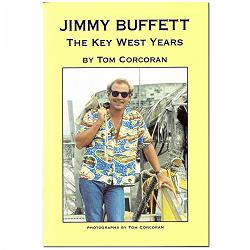The image depicts the cover of a book titled "Jimmy Buffett: The Key West Years" by Tom Corcoran. The cover features a small central photograph bordered by a light blue frame against a yellow background with blue text. The photograph portrays a white man, likely Jimmy Buffett, approximately 30 to 40 years old, with short, blond hair that's slightly receding. He's wearing dark sunglasses, blue jeans, and a short-sleeved, button-up Hawaiian shirt with the top two buttons open, revealing a necklace. He holds a jacket over his shoulder and is leaning on a boat dock railing. The bottom of the cover credits the photograph to Tom Corcoran.